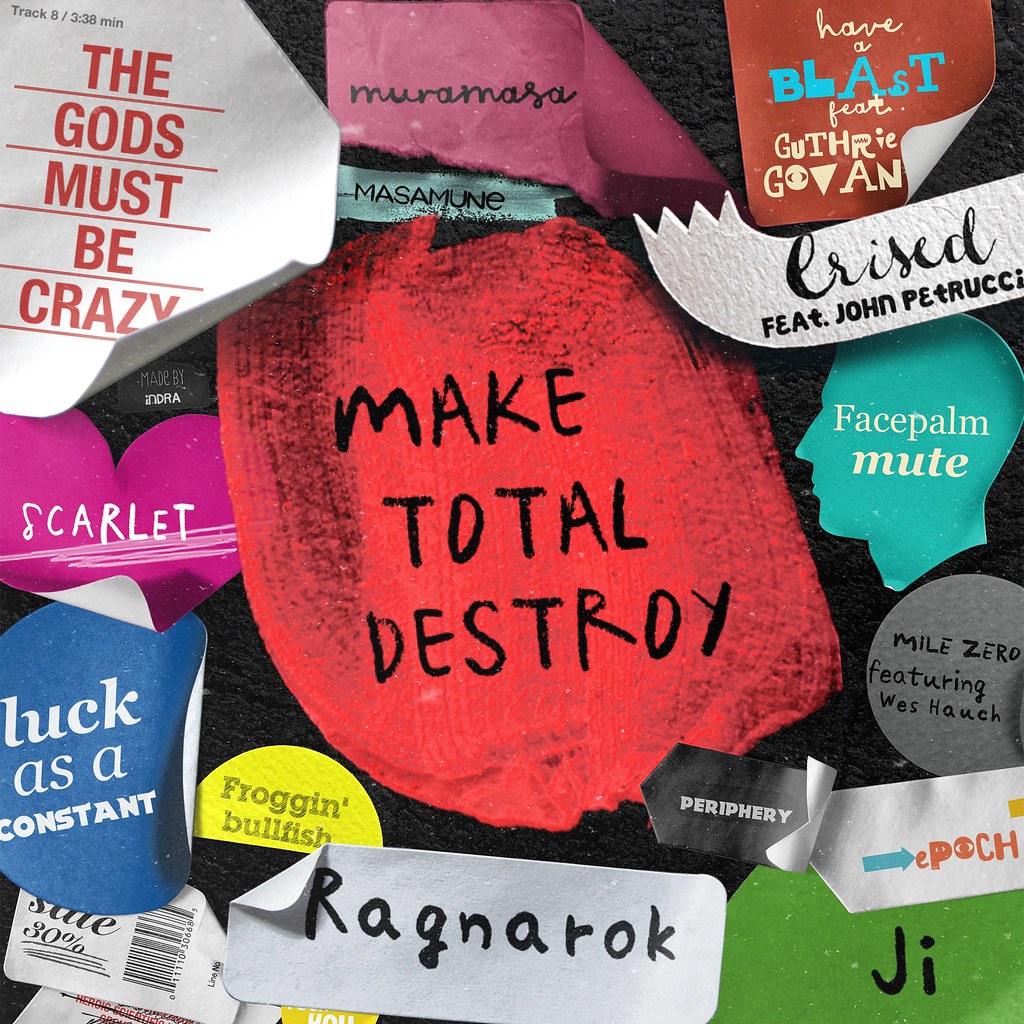The image is a collage resembling a black chalkboard covered with an eclectic mix of colorful labels, heart shapes, and circular paper cutouts that evoke the feel of stickers or Post-it notes. These vibrant pieces feature various titles and phrases as if haphazardly attached. On the top right, a white label with bold red text reads, "The Gods Must Be Crazy," reminiscent of the movie title. Below it, there’s a pink heart with the name "Scarlet," and a blue circle peeling away with the phrase "Luck as a Constant." A half-yellow, half-gray circle displays the words "Froggen Bullfish," while a white label with a peeling corner reads "Ragnarok." Prominently in the center, a red piece with black text declares "Make Total Destroy." Scattered around, various other colorful labels include titles like "Mile Zero featuring Wes House," "Facepalm Mute," and "Ragnarok," among others. The overall arrangement gives the impression of a vibrant, skater-boy aesthetic, possibly a page from a magazine, a folder, or even a book cover.